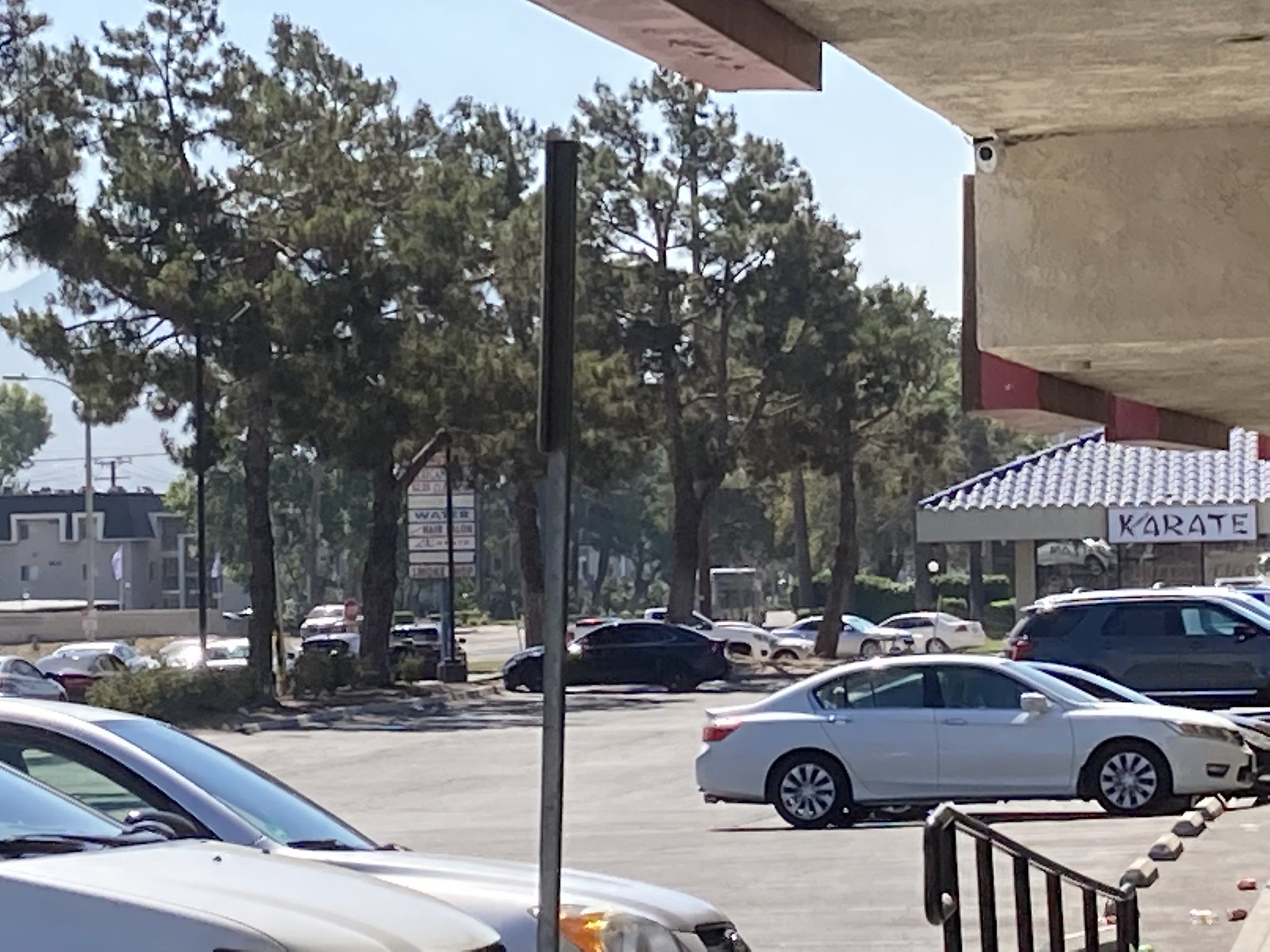The image captures a vibrant daytime scene in a parking lot under a clear blue sky. The lot is lined with a variety of vehicles, including several minivans and cars in colors such as white, gray, black, red, and silver. Prominently displayed is a white sign with black letters reading "Karate," attached to a structure with a white roof. In the upper left-hand corner, a surveillance camera is mounted on the wall, likely monitoring the parking area. 

Adjacent to the parking lot, a black railing lines the sidewalk, which is littered with discarded items like cans and cups. Across the street stands an apartment building, distinguishable by a flag hanging from one of its units. Streetlights and an array of telephone and electricity poles can be seen in the background, adding to the urban atmosphere. Overall, the image provides a detailed glimpse into a typical outdoor urban parking area shared by local businesses and residential buildings.